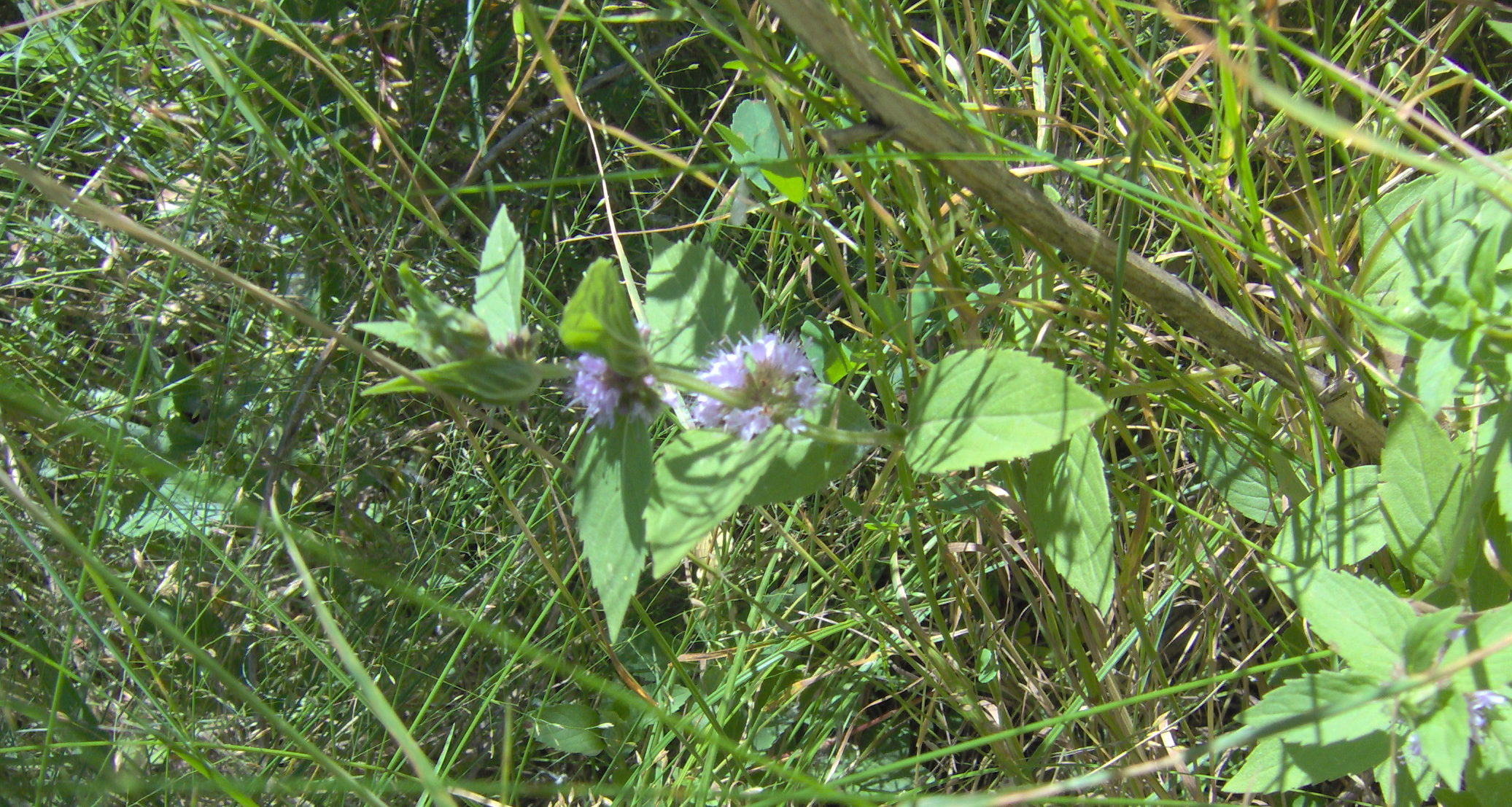This close-up photograph captures the natural beauty of an outdoor scene, likely taken midday under clear skies. The primary focus is a budding bluish-purple flower, positioned center frame, flanked by wispy petals. The flower is surrounded by an abundant mix of green leaves and long, unkempt grass. Among the greenery are several twigs and light brown branches, one of which extends from the right side towards the center-top of the image. Sunlight bathes most of the scene, illuminating the textures and colors, while a few darker, shaded areas are visible in the upper left. Additional smaller purple buds can be spotted across the scene, adding splashes of color to the verdant background. The overall composition gives a vivid glimpse into the untamed beauty of a natural field, brimming with life and subtle details.